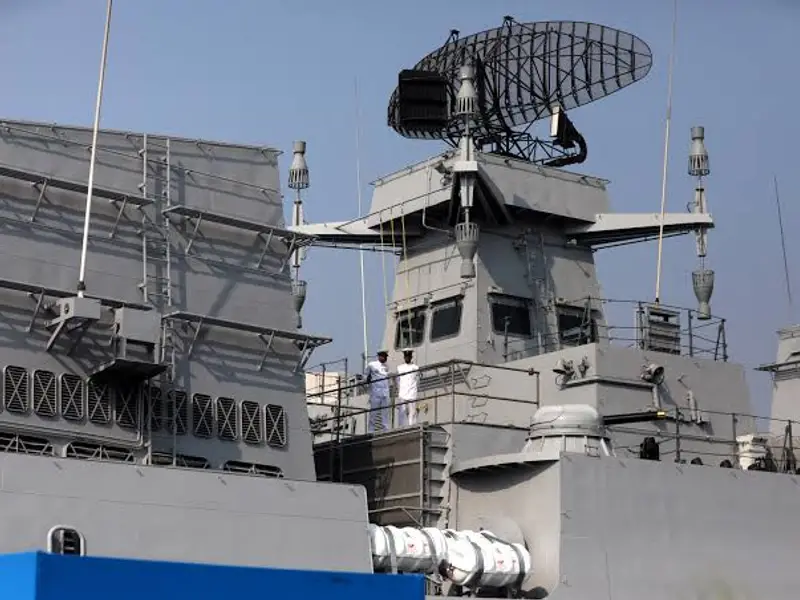This is a photograph of a naval battleship taken during the daytime against a muted blue sky. The image focuses on the middle section of the ship, which is predominantly light gray in color. Dominating the upper portion of the frame is a tower supporting a large, black radar detector that resembles a sideways oval mesh structure. The radar is facing away to the right side of the image. Two sailors in typical white naval uniforms, complete with caps, are positioned centrally on one of the upper decks. The deck is cluttered with various metal instruments and equipment, affirming its military nature. Below the deck, a prominent black pipeline runs along the nearest edge, and a rectangular dark blue object is visible in the foreground. Off to the left side, there appears to be a gray structure with windows, each reinforced with a giant metal X. The overall scene is grounded and complex, highlighting both human and technological elements of naval machinery.